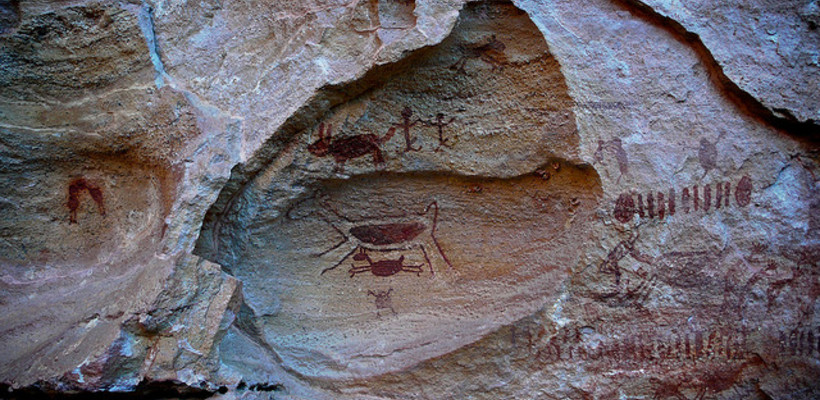The image depicts an ancient cave painting sprawled across the face of a massive rock wall with jagged cuts and sides. The rock itself is predominantly gray with patches of white and tan. The artwork, rendered in a brownish-red hue reminiscent of dried blood, features various crude illustrations. Prominently, there are depictions of four-legged animals, possibly horses, with a larger animal above and a smaller one, perhaps a juvenile or another similar creature, below it. Two stick-figure humans appear in pursuit of another four-legged animal. Additional stick figures, lines, and shapes are faintly visible to the right of the main illustrations, although they are difficult to discern clearly. The entire scene suggests a narrative or a hunt, captured in this ancient, primitive artistry.